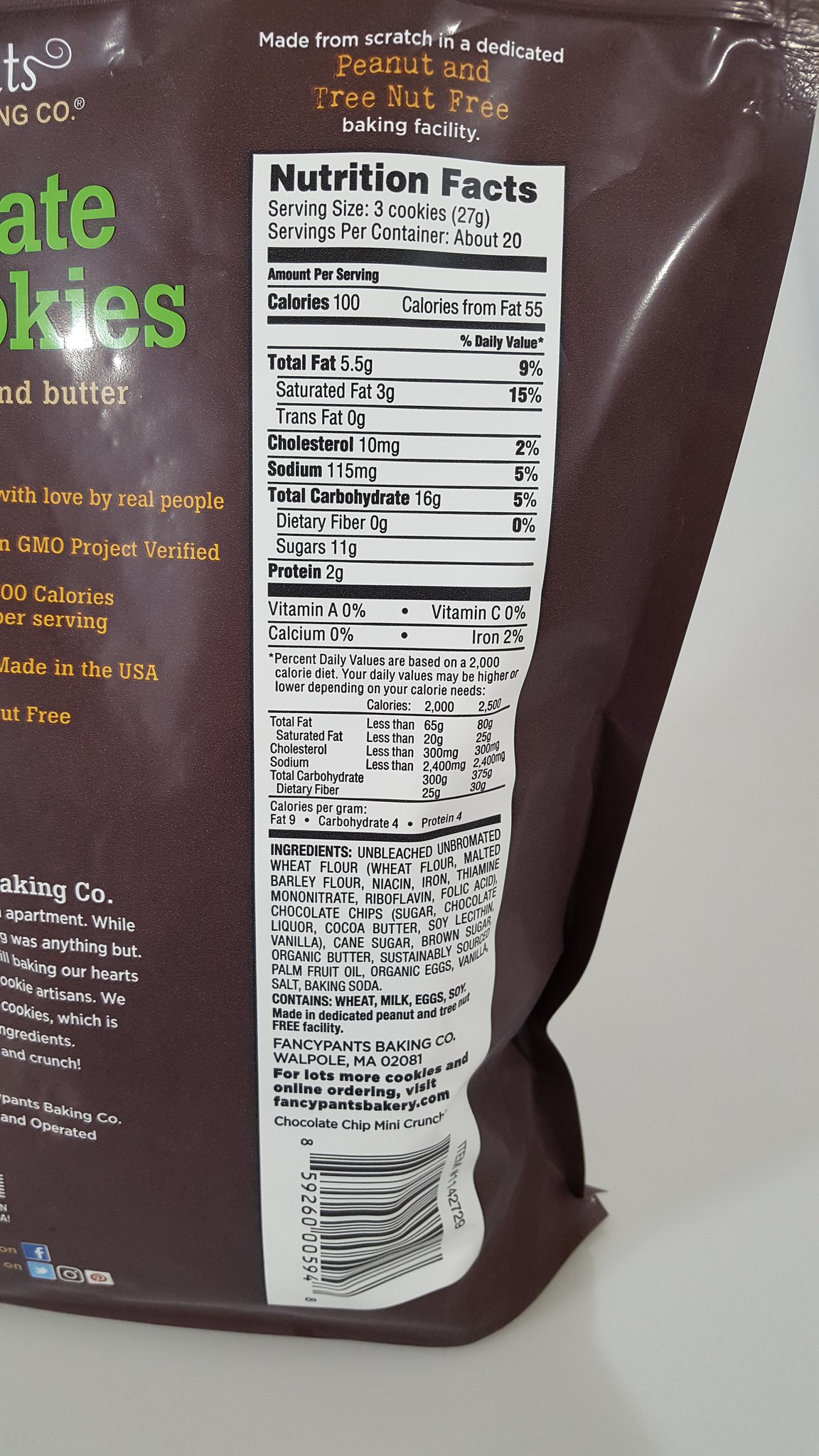This is a well-illuminated color photo of a chocolate cookie package positioned on a reflective, white countertop or tabletop. The reflection of the bag can be seen on the glossy surface, adding depth to the image. The package is predominantly brown, similar to the classic M&M's bag color, with sections of the package partially cropped out of the frame. The visible text on the bag indicates that the cookies are "made from scratch in a dedicated peanut and tree nut free baking facility." 

Prominent on the right side (though partially cropped) is the Nutrition Facts label, displaying detailed nutritional information: serving size is three cookies (28 grams), and the package contains about 20 servings. Each serving provides 100 calories, with 55 calories from fat. The total fat content is 5.5 grams (9% of the daily value), including 3 grams of saturated fat (15%), and 0 grams of trans fat. The cholesterol content is 10 milligrams (2%), sodium is 115 milligrams (5%), total carbohydrates are 16 grams (5%), and there are 0 grams of dietary fiber and 11 grams of sugars. The protein content is 2 grams per serving. The label also lists 0% for both Vitamin A and Vitamin C, 0% calcium, and 2% iron.

Other discernible details include partial text suggesting ingredients like "almond butter" and assurances like "GMO Project Verified" and "made in the USA." The label states that the product is created with love by a baking company located in Walpole, Massachusetts. The bottom of the package features a UPC barcode.